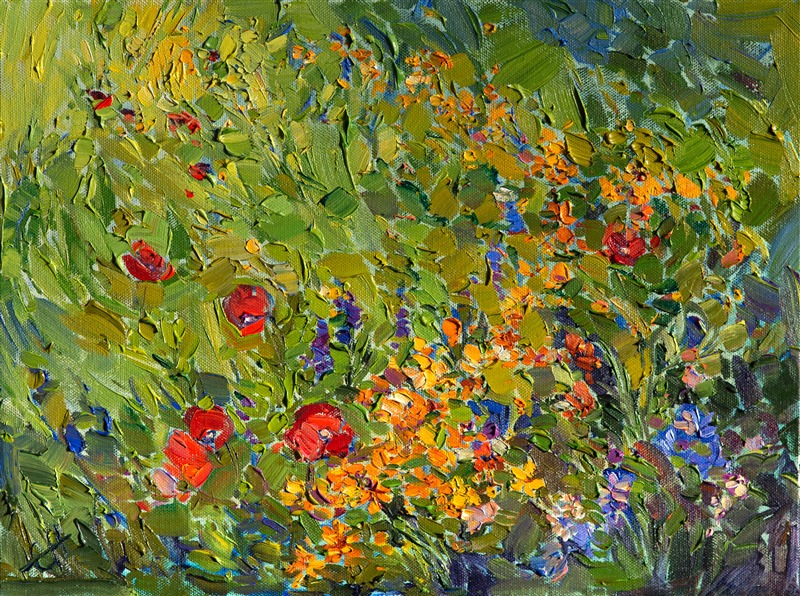The image showcases an Impressionist-style oil painting, characterized by its thick, textured brushstrokes and splotchy applications of paint. The painting vibrantly depicts a dense garden scene dominated by various shades of green, representing leaves and foliage. Throughout the canvas, there are striking speckles and patches of flowers in vivid hues of orange, yellow, red, purple, and blue. The composition reveals a concentration of florals beginning in the bottom right corner, becoming less dense as they dissipate upward. While the upper right quadrant of the painting is darker with more leaves and fewer flowers, the overall image is a beautiful and richly colored depiction of a garden, with no text present. The detailed brushwork and lush palette make it a visually engaging piece.